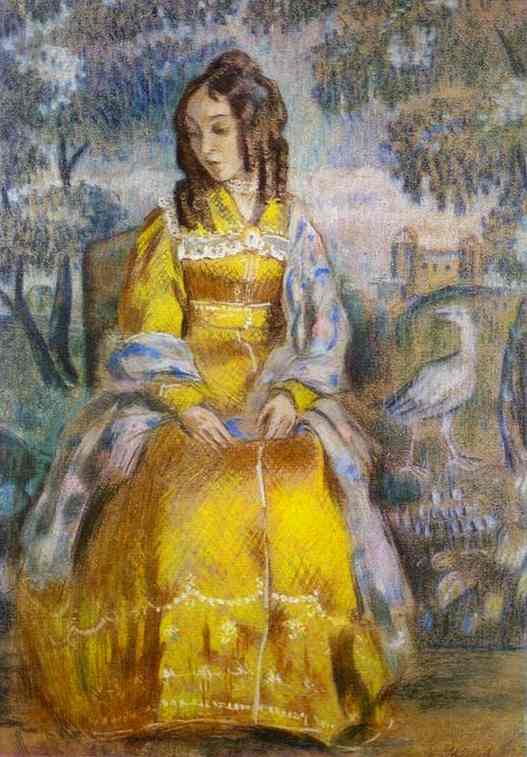This artwork is an impressionistic painting featuring a seated woman as its central subject. She is dressed in a floor-length, yellow gown with white chiffon trim, and a grayish-blue and yellow shawl draped over her shoulders and arms. Her brown hair is styled in long, curled locks that reach below her neckline, and she gazes downward to her right, giving an impression of contemplation. She is seated on a chair, hands resting gently on her lap. To her right stands a white bird. In the background, a scenic landscape unfolds with a house depicted alongside what appears to be a castle, flanked by lush, leafy trees. The painting employs a palette of yellow, green, blue, and white, capturing the scene in a somewhat impressionistic manner.